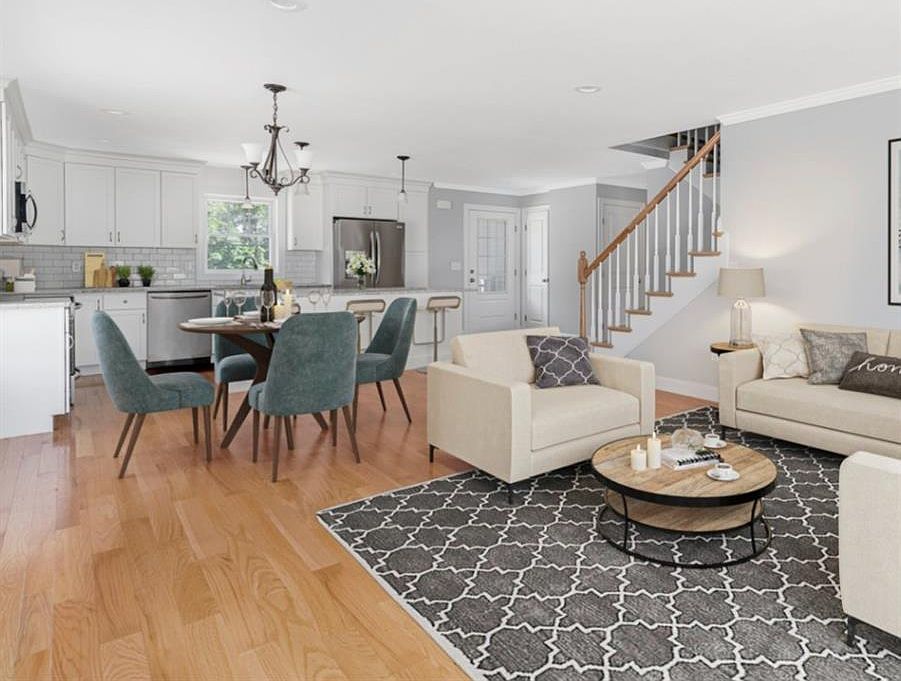This photograph captures an elegant open-floor-plan interior of a house that seamlessly integrates the living room, dining area, and kitchen. As you step inside, you're greeted by beautiful muted gray walls that create a soothing backdrop for the space. The kitchen, which lacks dividing walls, showcases modern white cabinetry and stainless steel appliances, including a dishwasher, stove, microwave, and refrigerator. At its center is an island area suitable for casual dining. 

Adjacent to the kitchen, there's a round dining table set for a cozy meal with candles and wine glasses, surrounded by four chairs which vary in descriptions from dark gray to blue to light green. This table area transitions effortlessly into the living room, where a light tan, almost cream-colored L-shaped couch and two additional chairs create a comfortable seating arrangement. The seating is centered around a round coffee table, either light or dark wooden with a distinctive presence, placed on a stylish gray carpet with white square patterns. Decorative pillows, a clear lamp on a side table, and partial views of a picture frame accent the sitting area, enhancing the welcoming atmosphere.

The polished medium dark-stained wooden floors shine brightly, leading towards a visible staircase with a brown railing that ascends to the second floor. The photograph also includes an entryway door situated near the kitchen, contributing to the functional and aesthetic flow of this inviting open space.